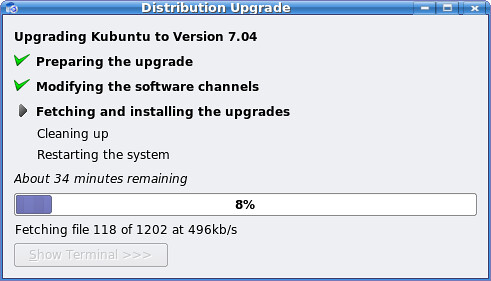The image is a vivid and detailed screenshot of a program window displaying a distribution upgrade for Kubuntu to version 7.04. The window sports a grey rectangular interface encased by a prominent blue border. At the top, white text announces "distribution upgrade," and familiar Windows icons for minimizing, maximizing, and closing the window are positioned in the upper right corner.

In the main body of the window, there is black text that tracks the upgrade process with specific stages: "upgrading Kubuntu to version 7.04," "preparing the upgrade" with a green checkmark, "modifying the software channels" with another green check mark, and "fetching and installing the upgrades" marked by a black arrow. Subsequent stages, "cleaning up" and "restarting the system," follow in regular font. 

Below these steps, italicized text estimates the time remaining: "about 34 minutes," and an extensive white progress bar fills partially with purple, indicating an 8% completion rate with a bold black number in its center. Beneath the bar, black text details the current file retrieval status: "fetching file 118 of 1202 at 496 KB/s." At the bottom of the window, a faded and unselectable box reads "show terminal >>>."

The overall color scheme includes blue for the percentage bar, black for the primary text, white for the background, and green for the checkmarks, all arranged logically from left to right. This configuration clearly indicates real-time progress and time estimation to the user during the upgrade process.